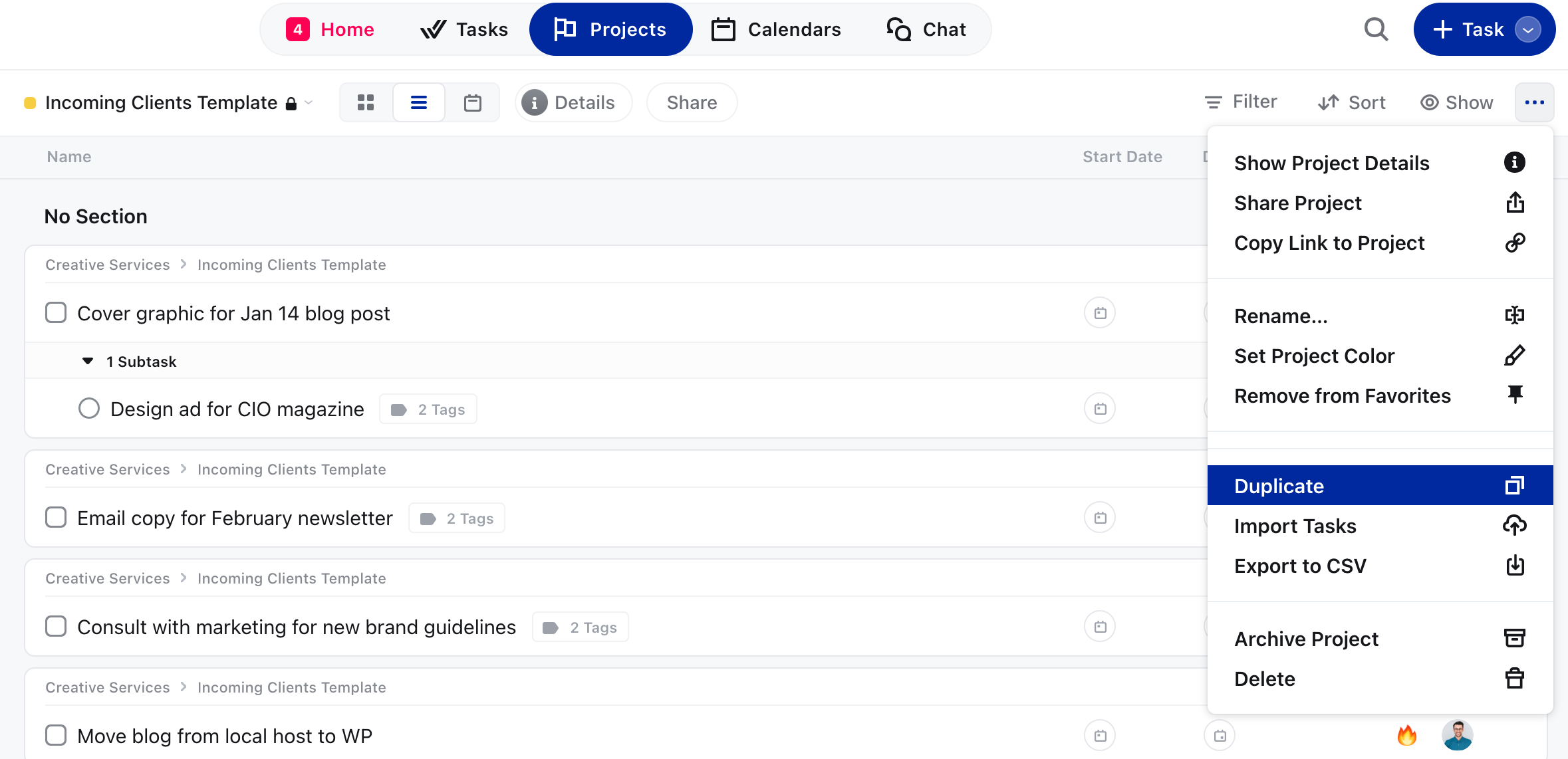Screenshot of a project management website interface. The navigation bar at the top features tabs labeled Home, Tasks, Projects, Calendars, and Chat, with the "Home" tab highlighted in red, indicating the active section. The "Projects" tab is displayed with a blue background, showcasing its importance.

Below the navigation bar, the "Projects" section is open, displaying an "Incoming Clients" template. The template includes detailed fields such as Name, Start Date, and Share options. Towards the upper right corner, there is a search icon represented by a magnifying glass.

Additionally, a blue rectangular button with a plus symbol and the word "Task" in white is prominently featured, indicating an option to add new tasks.

A pop-up menu appears with a list of actions available for the project. Options include "Show Project Details," "Share Project," "Copy Link to Project," "Rename...," "Set Project Color," "Remove from Favorites," "Duplicate," "Import Task," "Export to CSV," "Archive Project," and "Delete."

The interface is designed to provide comprehensive project management functionality, enhancing organization and collaboration on various tasks and projects.